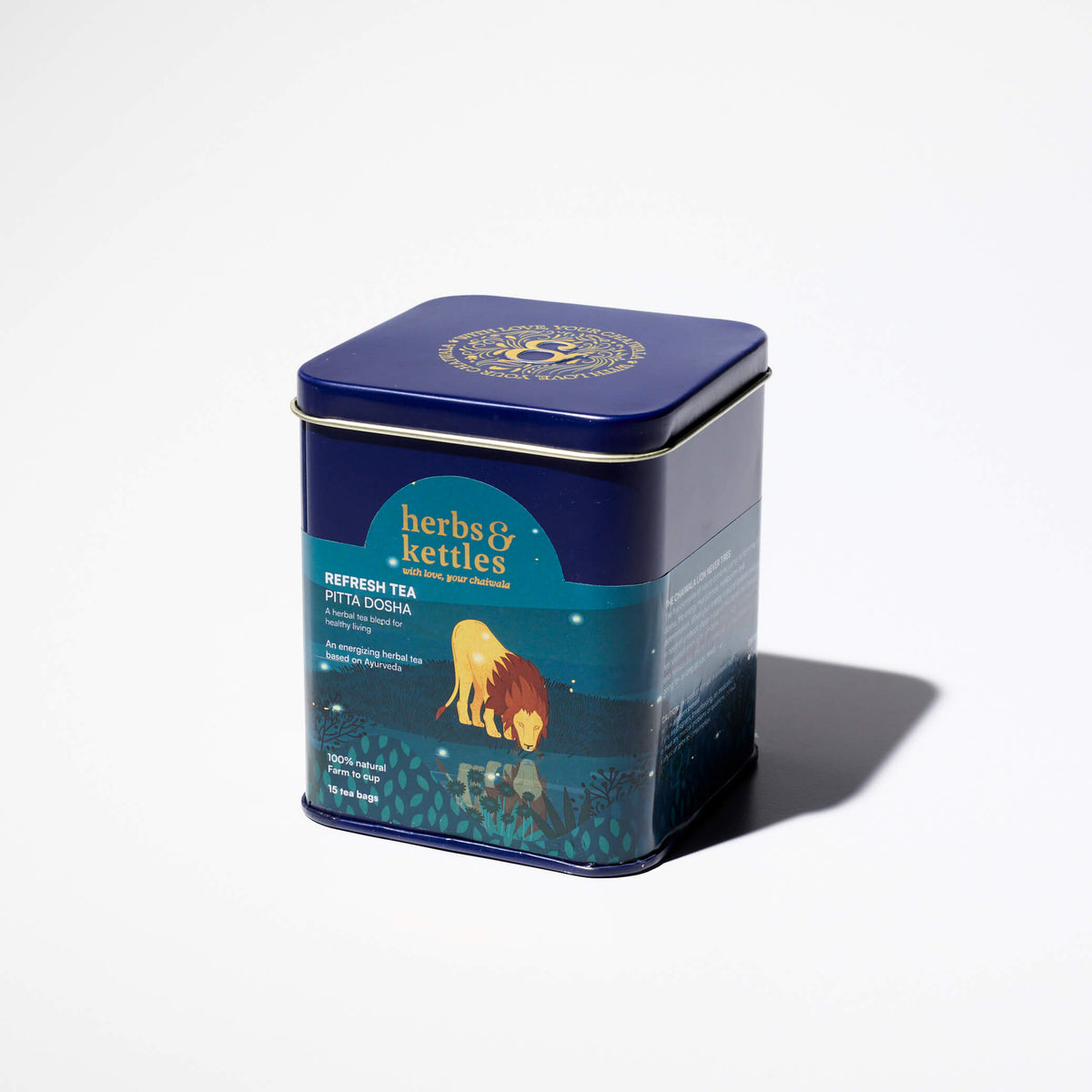The image features a square tin box labeled "Herbs & Kettles" designed for tea storage. The tin is dark blue with a teal front and silver edges around the lid. Prominently displayed on the front is an intricate illustration of a lion with a yellow body and a mane in shades of orange and brown. The lion is depicted drinking from a pond at night, with stars visible in the sky and its reflection mirrored in the water below. The tin is titled "Refresh Tea," indicating it is of the Pita Dosha variety. Additional details include the text "With Love" and mention of its 100% natural farm-to-cup tea, containing 16 tea bags. The entire scene is set against a stark white background, making the tin and its detailed artwork stand out.